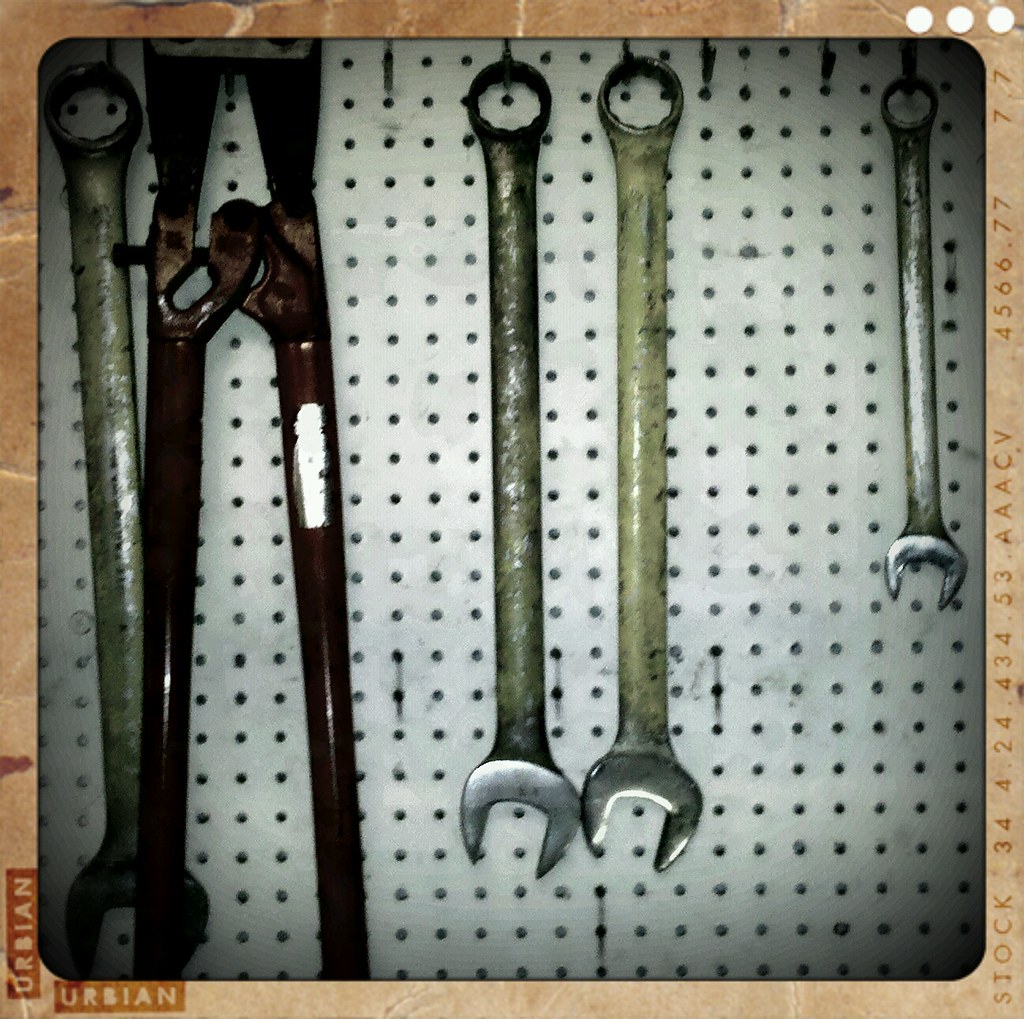This square photograph with rounded edges is set against a brown background that resembles a box or tiled area. The photo itself has digitally added borders, with the word "Urbian" in red and white text in the bottom left and a string of text "Stock 34424434 AAACV 4 56-6-77-7-7" running vertically along the right edge. In the top right corner, there are three distinctive white dots.

The central image depicts a greyish, perforated pegboard, characteristic of workshop or garage settings, with various rusted tools hanging from hooks. Starting from the left, there are several wrenches of varying lengths and conditions. The longest wrench, positioned to the far left, has a greenish, rusted appearance. Next to it, partially cropped out of the picture, is a set of bolt cutters with dark red handles. Further to the right, two more wrenches follow, sharing a similar yellowish-green hue indicative of rust. Finally, on the far right, a smaller, relatively pristine silver wrench reflects light and hangs alone. In the middle of the pegboard, three hooks are empty, adding to the utilitarian aesthetic of the composition.